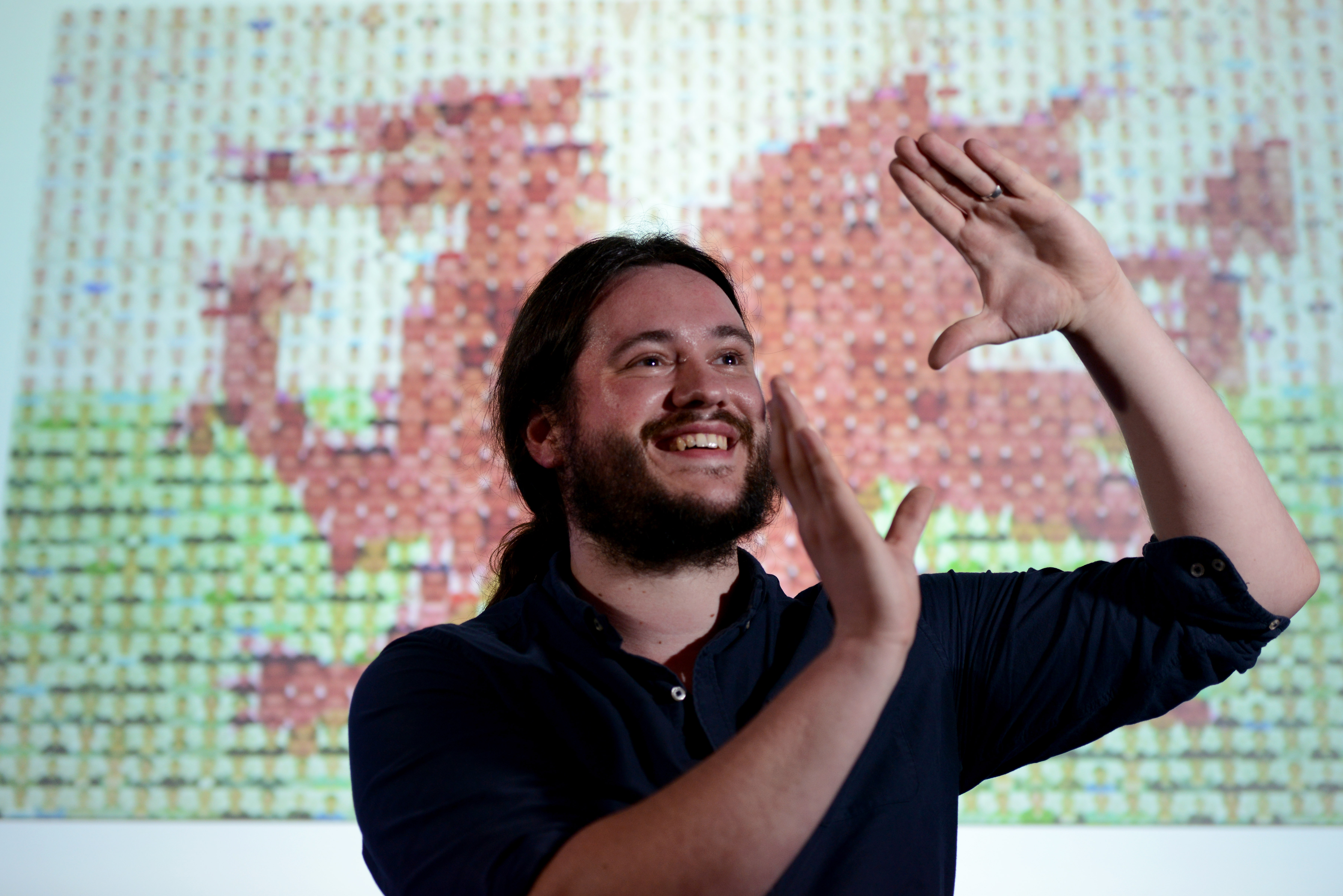The image depicts a smiling, bearded man with long, dark hair tied back in a ponytail. He is wearing a dark blue, long-sleeved, button-up collared shirt with the sleeves pushed up to his elbows. His hands are raised and positioned as if he's framing a shot or looking through a viewfinder. Behind him, the wall features a light blue horizontal strip, and above it hangs a colorful, pixelated artwork. The artwork appears to depict a red dragon on a multicolored, somewhat blurred background with various hues of yellow, blue, green, and white lines. The man is looking slightly to his left, adding to his cheerful demeanor in the scene.